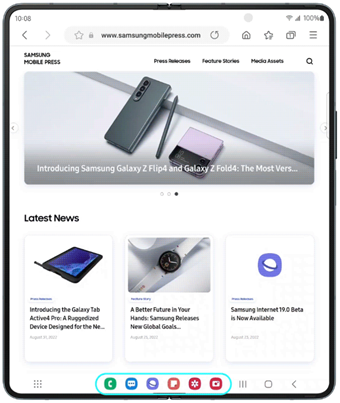A detailed caption for the described image might be:

"A high-resolution mock-up showcases a user interacting with an app on a Samsung hinged smartphone. The device, notable for its black edges and clearly visible buttons, features a hinge running down the center, suggesting it is one of Samsung's foldable models. The screen displays the 'Samsung Mobile Press' website, identifiable by the URL 'samsungmobilepress.com' in the browser toolbar. Icons are rendered crisply at 100% scale. The webpage's hero section advertises the 'Samsung Galaxy Z Flip 4' and 'Galaxy Z Fold 4' with an image displaying the phones – one with a stylus and the other folded like a flip phone. Below the hero image, there's information divided into three tabs. The first tab announces the 'Galaxy Tab Active 4 Pro,' a ruggedized device, though part of the description is obscured. The second tab features a smart watch and highlights new global goals, while the third tab mentions the 'Samsung Internet 19.0 Beta' availability. The bottom of the screen shows a teal-colored capsule highlighting various icons like a phone, text, planet, documents, and gear, each color-coded in green, blue, purple, orange, and shades of red. This highlight appears to be part of the visual design rather than functional elements of the actual website."